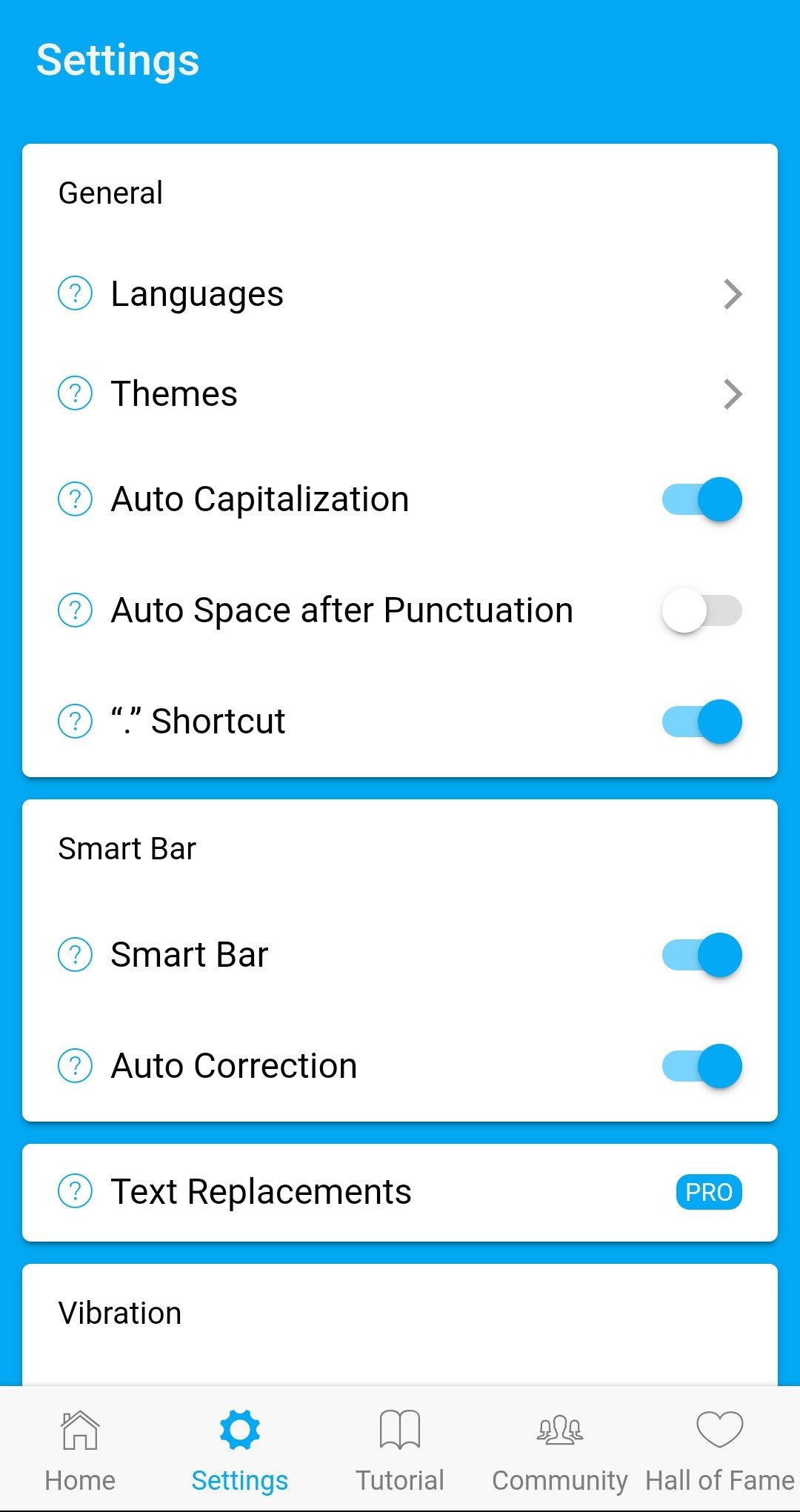On a predominantly light blue background, the image highlights various settings in a clear, organized format. At the top left corner, the word "Settings" is prominently displayed. Below that, a white rectangular section titled "General" is visible. 

Within this section, several options are listed:
1. To the left, an icon consisting of a blue circle with a question mark inside is labeled "Languages," followed by a right-pointing arrow.
2. Next, another blue circle with a question mark labeled "Themes," accompanied by another right-pointing arrow.
3. Another option labeled "Auto Capitalization" follows a blue circle icon.
4. Below this is a setting for "Auto Space After Punctuation" displayed with a light blue bar and a dark blue circle, and another question mark icon.
5. Further down, "Quote, Period, Unquote Shortcut" is represented by a blue circle and a bar.

A blue space separates the next section labeled "Smart Bar," which appears in another white rectangle. Here, the icon with a question mark and a circle reappears, labeled "Smart Bar," followed by a light blue bar and dark blue circle. Below this, "Auto Correction" possesses a similar layout with a blue bar and dark blue circle.

Further down, another white rectangle is labeled "Text Replacements," accompanied by the familiar circle with a question mark. Adjacent is a blue rectangle with curved corners marked "Pro."

At the bottom, the top of another white rectangle is visible, showing a setting for "Vibration." Below is a light gray rectangle featuring several icons: 
- A house with the label "Home"
- A blue gear icon under the label "Settings"
- An open book icon labeled "Tutorial" in gray
- People icon labeled "Community"
- An outlined heart labeled "Hall of Fame."

Each icon is positioned neatly, indicating intuitive navigation and user accessibility.